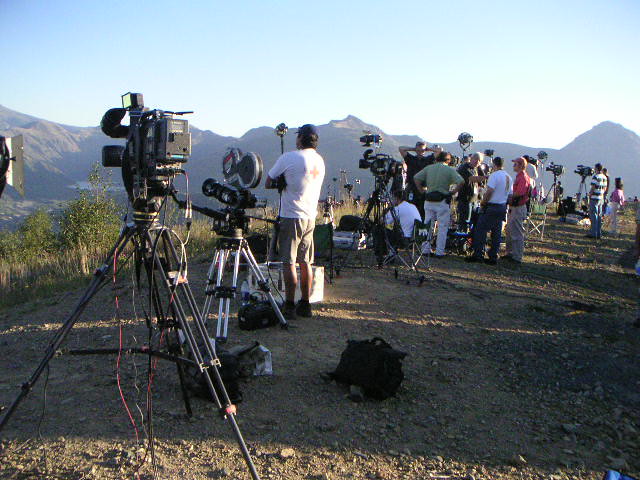The image captures a bustling movie set from the late 80s or early 1990s, situated on a dry, browns-toned hill overlooking a vast and arid mountain range. The sky above is a gradient of light to deep blue, sans any clouds, indicating it's early morning. In the foreground, there's a ledge scattered with stones and sparse, shrubby green plants. At least seven movie cameras on tripods, including traditional film cameras with reels, are lined up from the left side of the frame extending into the distance. Various teams of operators and crew members, mainly men, are either standing by the cameras, sitting, or huddled together in conversation. Close by, a man in a white t-shirt, cargo shorts, and sneakers prominently faces away from the camera, while a white-haired man in similar attire faces the lens in the background. The scene is littered with equipment bags, and a few crew members are adorned in hats or fanny packs, further validating the period. A speck of director's chairs is also visible amidst the congregation. The barren, sunlit mountain range in the distance underscores the dry, desert-like environment of the setting.